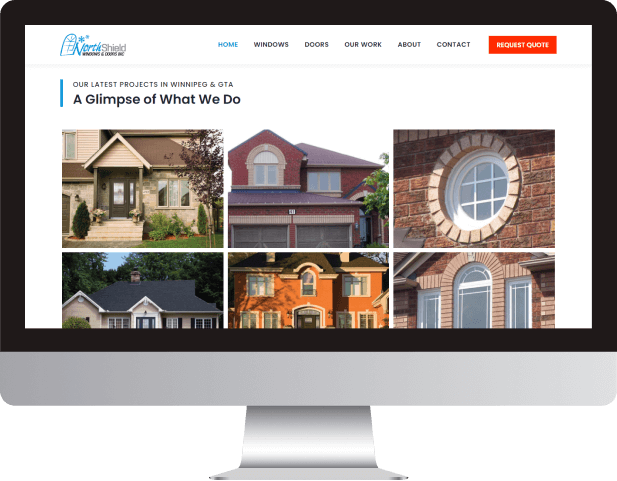The image showcases a computer monitor displaying a website. The monitor brand is not identifiable due to the lack of visible branding. The website in focus is titled "North Shield." The homepage features a distinct logo of a rounded-top window flanked by stars. The website navigation bar, located at the top, includes links to "Home," "Windows," "Doors," "Our Work," "About," and "Contact." In the upper right-hand corner, there is an orange button labeled "Request Quote."

Beneath the navigation bar, there's a heading that reads "Our Latest Projects in Winnipeg and GTA - A Glimpse of What We Do." Below this heading, a series of six images showcases various parts of residential houses. The first image features the front door, stairs, and a single window of a tan-colored house. The second image depicts a red brick house with two garage doors and two windows situated above them, with one on the left and one on the right. The third image focuses on a round window framed in tan and set in a brick wall, featuring window dividers. The fourth image predominantly shows the roof and upper windows with trees visible in the background. The fifth image presents an orangey-red house showing the front door and multiple windows. The last image captures an arched window flanked by two side windows set in a brick house.